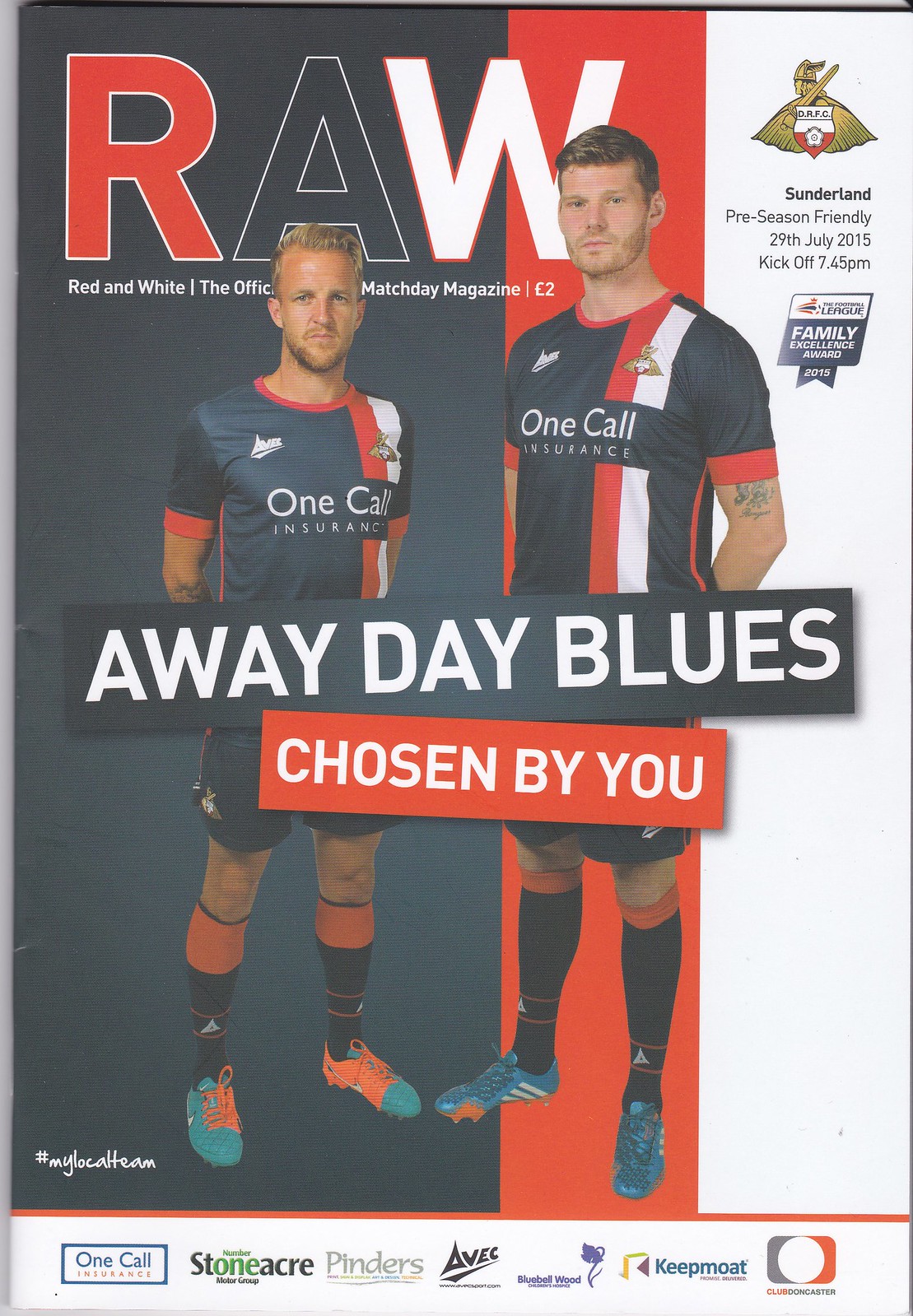This is a scan of the cover of a soccer program titled "R.A.W.", with each letter in red, navy, and white respectively. Below the title, in smaller white text, it says "Red and White, The Official Matchday Magazine" along with a price tag of two euros. The background features thick blue vertical stripes alternating with thinner red and white vertical stripes. At the top right, there's a club crest and information about the match: "Sunderland Preseason Friendly, 29th July 2015, Kickoff 7:45 p.m." with additional details about a "League Family Excellence Award 2015."

Prominently in the center are two players, one with blonde hair and a beard and the other taller with light brown hair and a five o'clock shadow, both wearing blue, red, and white vertically-striped jerseys with the sponsor "OneCall Insurance" on the front. The cover's tagline is displayed across a navy bar and a red bar in all caps white text: "AWAY DAY BLUES, CHOSEN BY YOU." At the bottom, there's a white strip containing various sponsor logos including Keap Moat, Avec, and OneCall. Additionally, a white hashtag "#MyLocalTeam" is visible, contributing to the community feel of the publication.